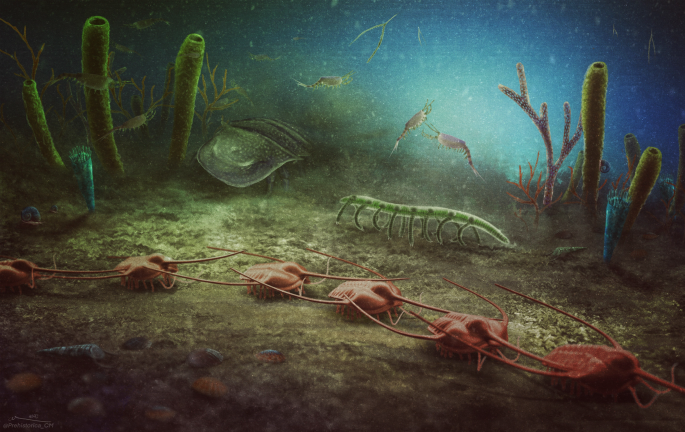The image is a rectangular, computer-generated illustration depicting an underwater scene. In the foreground on the ocean floor, which transitions from dark gray at the bottom left and right-hand corners to a brown and light greenish-tan towards the center, a caravan of six reddish-toned crustaceans with hard armor-like backs, thin-pointed hooked noses, and long dangling antennae, march across the seafloor. These creatures have numerous legs, contributing to their distinct shellfish or crab-like appearance.

Behind this crustacean caravan, a long green centipede-like creature, featuring about 20 legs—10 on each side—and a translucent body is depicted, adding an eerie ambiance to the scene. The background hosts various elements, including tall conical tube plants that resemble cacti and are colored green. Among these plants, small fish and prawn-like creatures swim, and the water is filled with floating debris.

The illustration’s palette shifts from a light blue circular area in the upper right-hand corner, indicating a light source, to a darker blue, almost black, at the top edges. The setting is illuminated by this light source, creating a contrast with the darker stones scattered across the ocean floor. This detailed underwater tableau is further enriched by the presence of larger and smaller fish, adding life to this vivid marine ecosystem.